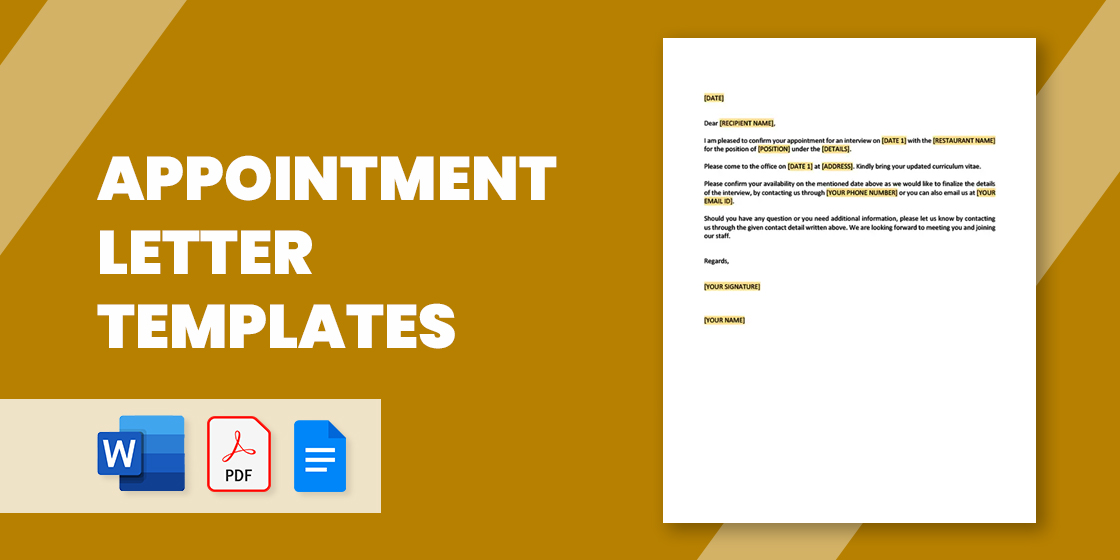The image showcases an "Appointment Letter Templates" advertisement set against a predominantly mustard-colored background with vertical tan stripes. Dominating the center-left, bold white text in all caps announces "APPOINTMENT LETTER TEMPLATES." Directly below this, three recognizable icons are aligned horizontally: a blue Rectangle with a gradient from light to dark blue featuring a white 'W', representing Microsoft Word; a white square with a red border and a stylized red 'loopy triangle' symbolizing PDF format; and another blue rectangle with three white lines associated with Google Docs. 

On the right side of the image, there is a detailed template letter. The template is a white, letter-sized document with several highlighted sections in an orange-yellow hue. These highlights indicate placeholders for personal information such as "dates," "recipient name," "position," "address," "your phone number," "your email ID," "your signature," and "your name." These placeholders are intended to be filled out by the user. The template begins with a greeting and moves on to confirm an interview, requesting the recipient to bring their updated curriculum and confirm their availability. The document concludes by expressing anticipation for the recipient's potential addition to the staff.

Overall, the image is a professional template offering with easily identifiable format options and necessary placeholders for customization, all set within a visually structured and color-coordinated background.